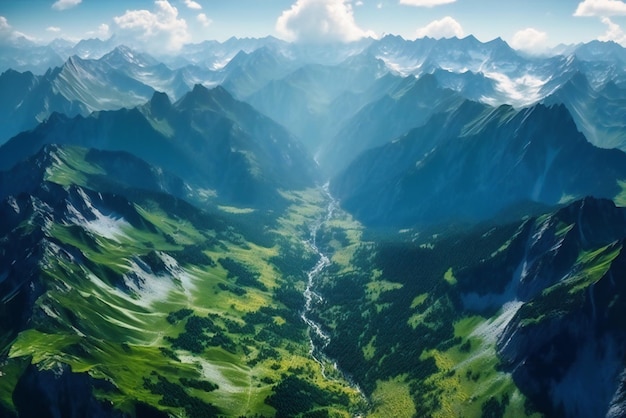This highly realistic digital illustration, resembling a photorealistic aerial photograph, captures a breathtaking mountain landscape. The focal point of the image is a narrow, zigzagging stream that trickles through a deep, lush valley, drawing the viewer's eye towards the vanishing point. Surrounded by towering, jagged peaks, the valley is a patchwork of vibrant green grass and dense trees, contrasting sharply with the dark green, craggy mountainsides. Patches of snow dust the higher altitudes, adding a sense of chill and elevation, much like a sprinkling of powdered sugar. The scene is bathed in the bright natural light of daytime, enhancing the vivid colors and crisp details. Above, the clear blue sky is adorned with fluffy, white clouds, completing this serene and idyllic depiction of a mountainous paradise.